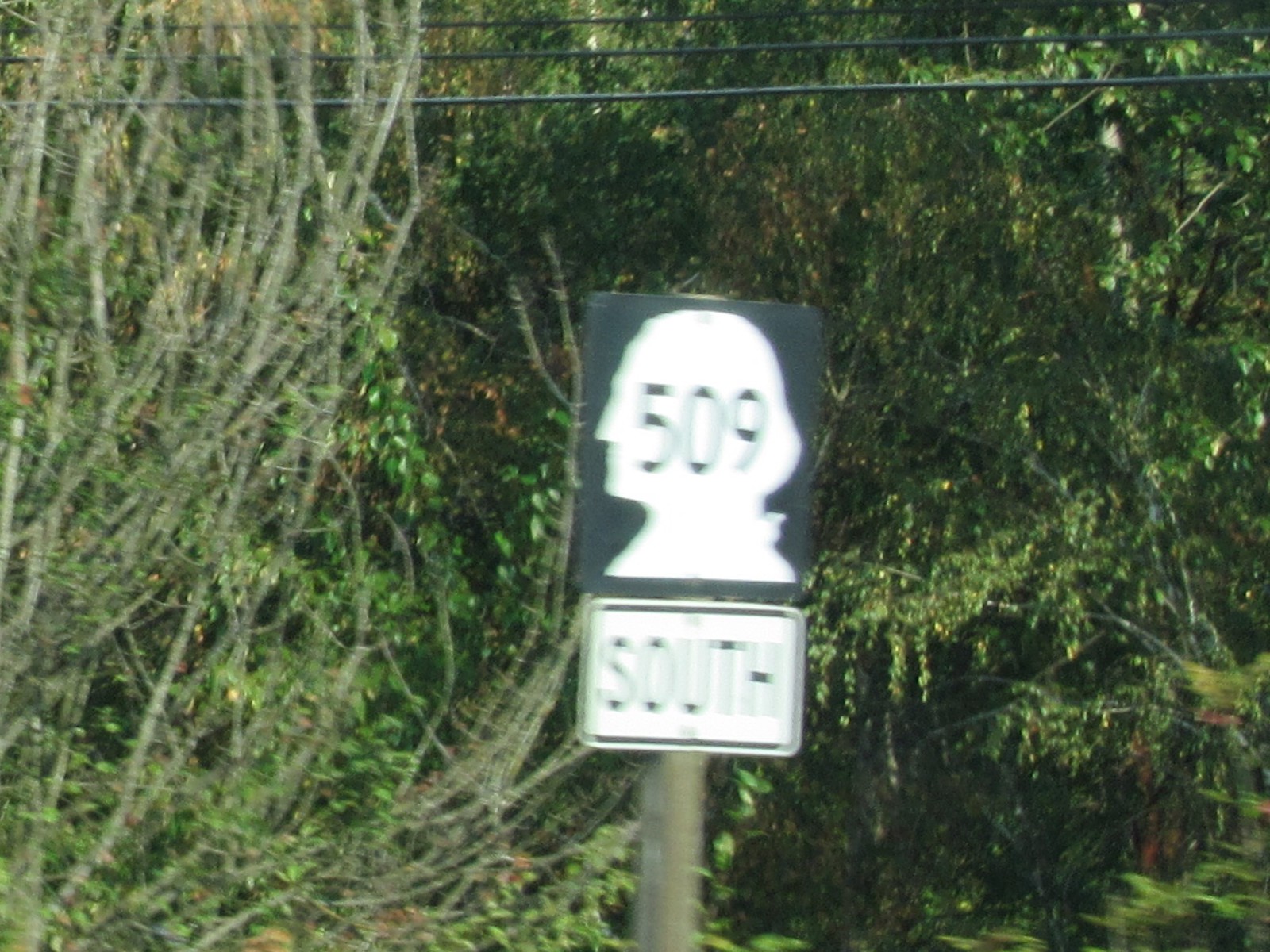This horizontal photograph captures a serene countryside scene, deeply immersed in lush greenery and natural beauty. Dominating the landscape are abundant trees and dense shrubbery that stretch out into the distance, giving the image a rich, vibrant texture. Above this verdant tableau, three black power lines traverse the upper portion of the frame, cutting horizontally across the sky, juxtaposing nature with a hint of human infrastructure.

Central to the foreground is a prominent road sign, which draws immediate attention. The sign is black with a striking white silhouette of George Washington at the top, and below it, a white rectangle with a black border surrounds the text. Displayed within Washington's silhouette is the number "509" in bold black characters, signifying a specific route. Directly beneath, in no-nonsense black letters, is the word "South," indicating the directional flow of this road. The sign is securely mounted on a round metallic post, standing firmly amidst the country setting. Interestingly, George Washington's profile on the sign faces or points to the left side of the image, guiding travelers forward.

Overall, this detailed composition intertwines elements of rustic charm and man-made direction, encapsulating both the tranquility of the countryside and the journey of the road.